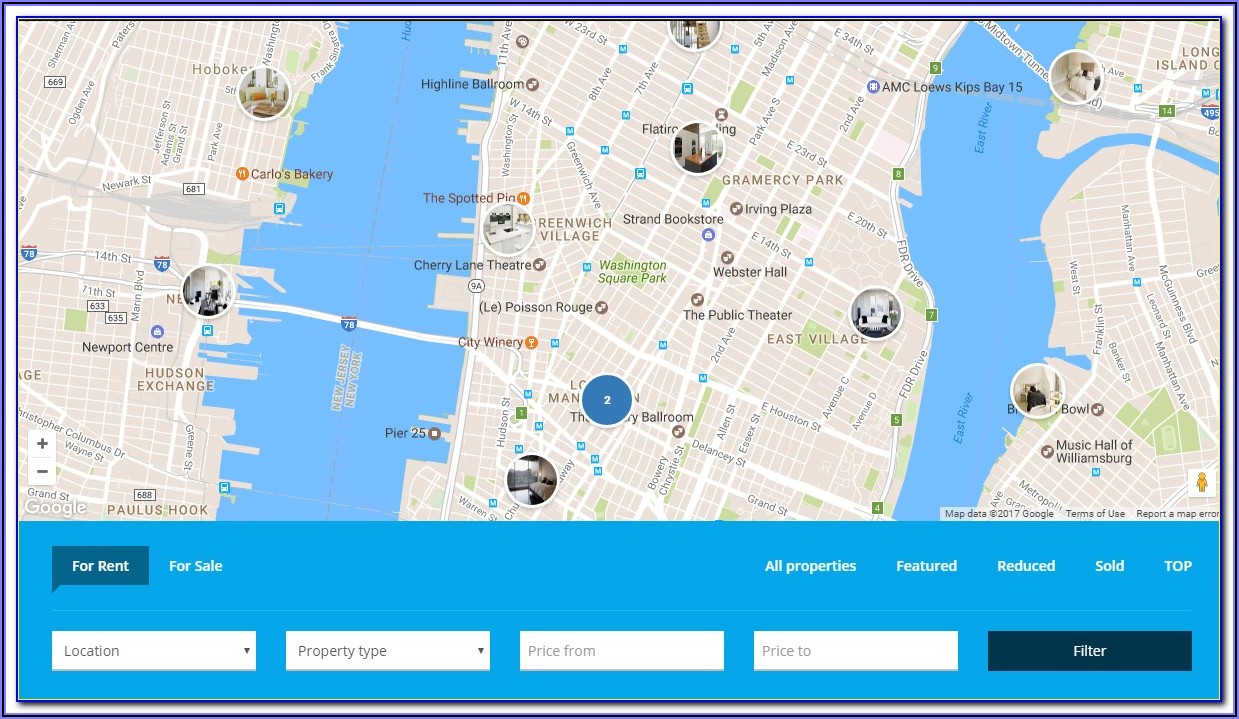This image captures a detailed map focusing on various neighborhoods and landmarks in New York and parts of New Jersey. The map is divided into three distinct sections. 

In the first section, notable areas include Newport Center, Hudson Exchange, and Paulus Hook, with prominent streets like Christopher Columbus Drive and Wayne Street visible. This segment also features a waterway and Interstate 78, which connects to the second section of the map.

The second section highlights key locations such as Webster Hall, Washington Square Park, Greenwich Village, Gramercy Park, AMC Loews, and East Village. This area is delineated by another water body, the East River.

In the third section, towards the top, the map includes the Midtown Tunnel, Long Island, and the Music Hall of Williamsburg.

Below the map, there is a row of categories labeled "All Properties," featuring sub-labels like "Feature," "Reduced," "Sold," and "Top." On the left-hand side, options for "For Rent" and "For Sale" are clearly marked. This suggests that the map is a digital interface for a real estate platform, allowing users to search for properties. The interface includes dropdown menus for selecting "Location," "Property Type," and setting "Price From" and "Price To" ranges. There is also a "Filter" button, prominently displayed in a dark box with white lettering, indicating a customizable search functionality to help users find properties within a specified price range.